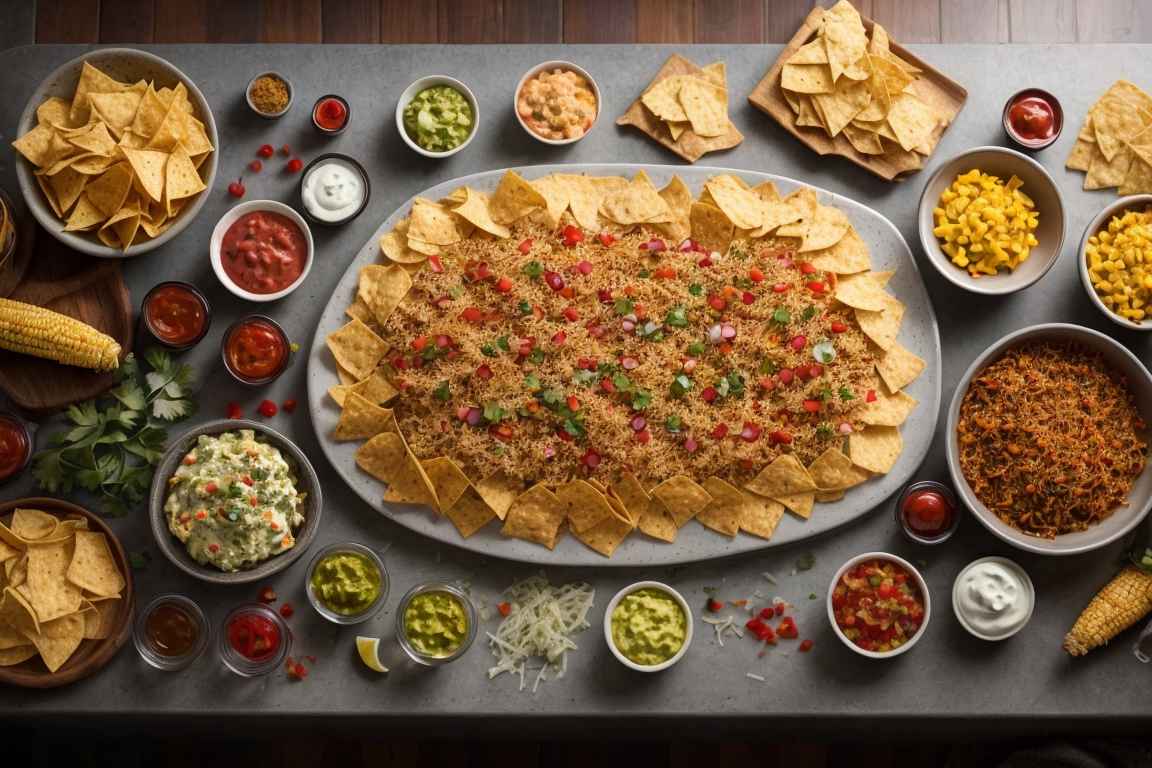The image depicts a rich, indoor tabletop setting featuring an elaborate spread of nachos and various accompaniments. The scene is centered on a large, slightly misshapen grey oval plate holding a heap of fried Mexican rice, topped with bits of pork, bell peppers, cilantro, possibly onions, and dotted with green and red garnish, likely scallions or tomatoes. This pile is encircled by a ring of crispy tortilla chips. Surrounding the main plate are an assortment of smaller bowls, each containing different toppings and sides including shredded meat, corn on the cob (in a brown bowl), guacamole, salsa, sour cream, ketchup, and mayonnaise.

The table itself is a blend of earthy and sleek elements—a gray table runner or countertop surface beneath the dishes, juxtaposed against the horizontal wooden slats of the brown table peeking from the top edge of the photograph. Additional bowls, potentially containing leafy vegetables, are scattered around, adding to the diversity of textures and flavors. This inviting and colorful setup suggests a "build-your-own-nachos" feast, set against the backdrop of a cozy, wood-floored indoor space.